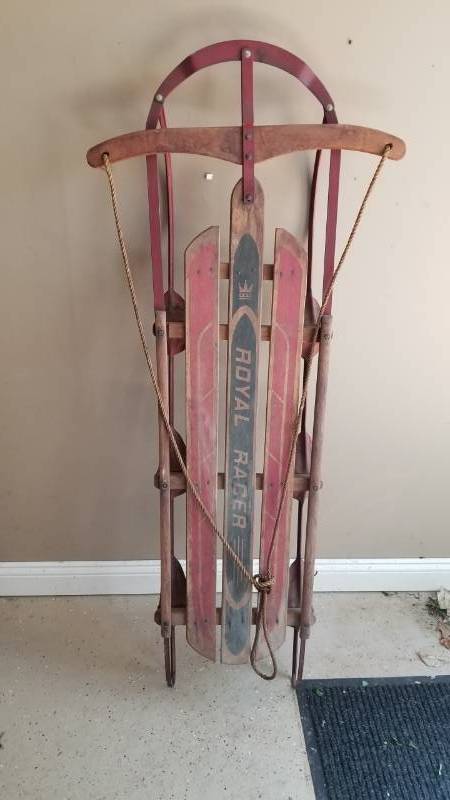The photograph features a well-used Royal Racer sled, showcasing its vintage style and robust design. The sled consists of a sturdy metal frame with three wooden slats for seating or laying down, painted red with black accents. Prominently displayed in the center is the "Royal Racer" label, crowned at the top. A steering rope, tied in a knot, extends from the top wooden slat. The sled is vertically propped against a beige wall with a white border, and a black mat lies on the dirty linoleum floor in front of it, adding context to its storage environment, which appears to be a garage. The image seems to be taken with a mobile phone, possibly for a sale listing, capturing the sled's nostalgic charm and utilitarian function.